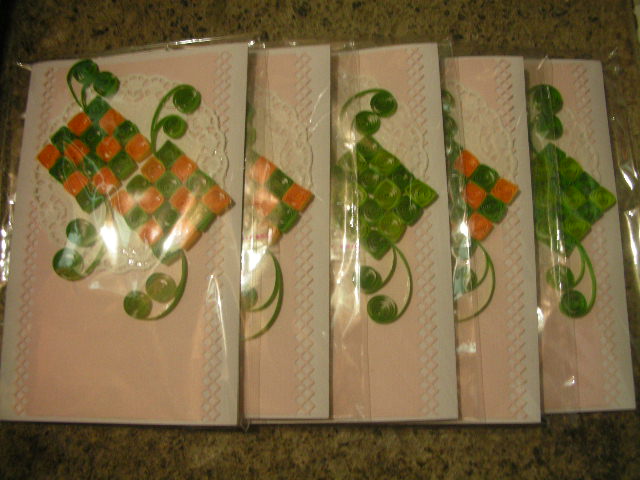The photograph, taken from a bird's eye view, shows a series of five horizontally aligned paper napkins, slightly overlapping one another, on what appears to be a granite or sandstone kitchen countertop. The napkins are individually sealed in thin plastic sleeves for sanitation. The first napkin on the far left shows a detailed design featuring two red and green checkerboard patterns inside diamonds, accented with a vine of greenery. Each subsequent napkin mirrors a similar pattern. The second napkin replicates the design of the first, the third shifts to an all-green checkerboard pattern, the fourth reverts to the red and green design, and the fifth and final napkin again features the all-green pattern. The overall look resembles a series of homemade cards, with intricate, marbled-like designs potentially made of fused beads or half-marble elements, predominantly in green and orange. Additional decorative elements like lace, doily patterns, and swirled greenery enhance the visual appeal, creating an impression of layered and detailed craftsmanship.